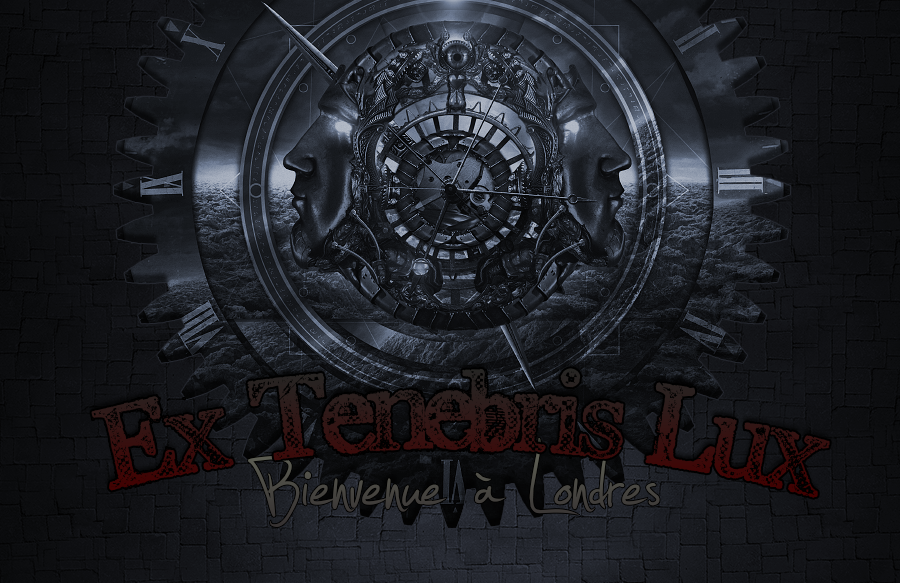The image features a dark gray or black background, with a hand-drawn gray brick wall texture at the bottom. Dominating the center of the image is a large, silver metallic disk resembling a gear, complete with spiked teeth around the edges. The gear features a sheen, with the sides mostly illuminated while the top and bottom parts remain in shadow. Inside the gear, a ring encircles an intricate design: two cyborg-like faces, one facing left and the other right, connected back-to-back and embellished with mechanical details above their foreheads and under their jaws. At the top of the gear is a hole, resembling an eye. Beneath this central illustration, in bold red letters, is the text "Ex Tenebris Lux," with each initial letter capitalized and displaying a gradient from rusty brown at the top to dark red at the bottom. Below this, in a lighter, casual font, are the words "Bienvenu à Londres." The combination of elements suggests a poster with a futuristic or dystopian theme.